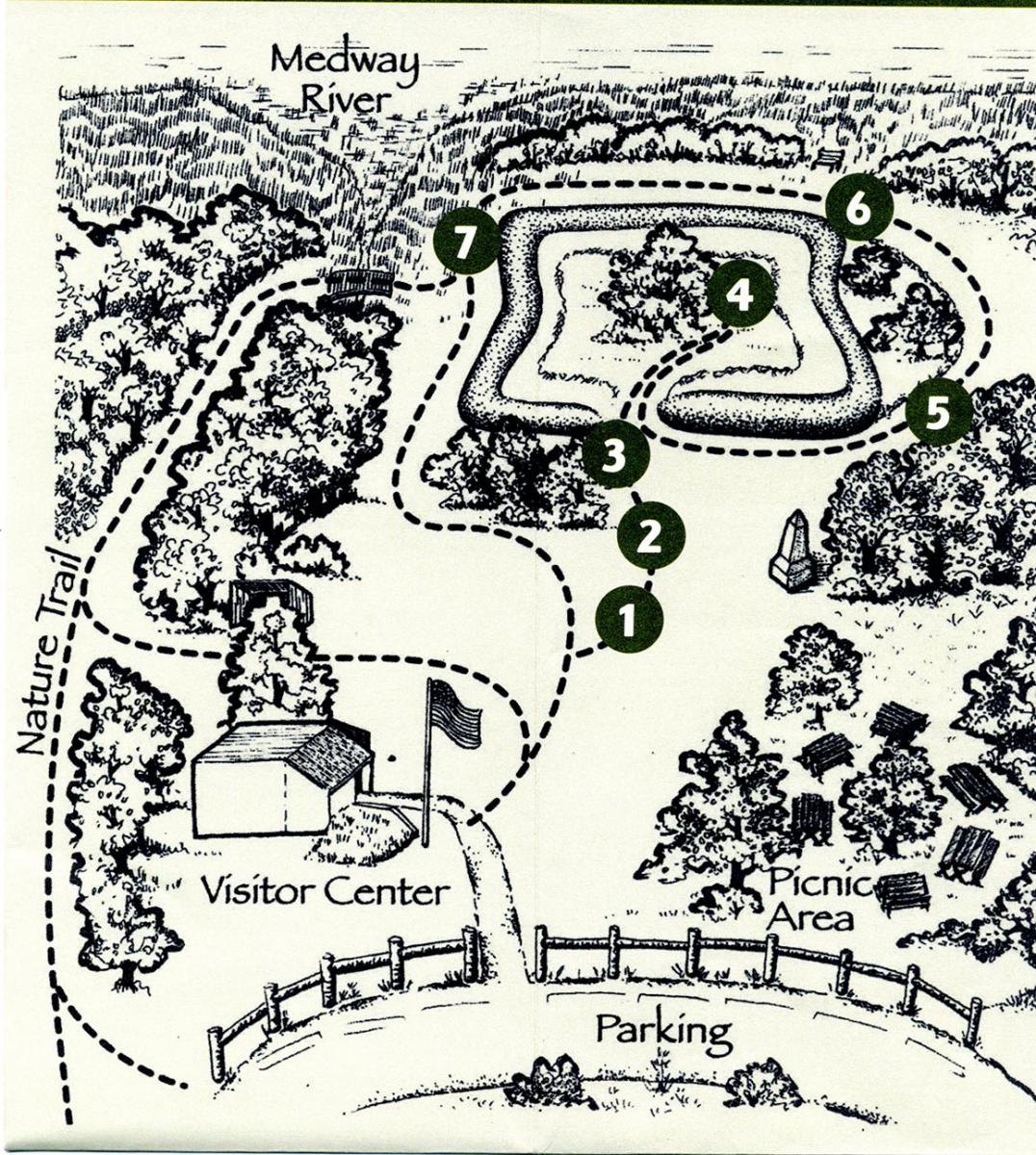This black and white aerial depiction illustrates a regional park adjacent to the Medway River, prominently located at the top of the image and encircled by lush green vegetation. Starting from the bottom, the map indicates a fenced parking lot leading to the main entrance. Directly to the left of this entrance lies the visitor center, distinguishable by the depiction of an American flag. To the right of the entrance, the picnic area occupies the lower right quadrant, featuring six picnic tables amid a dense cluster of trees. The park layout is marked by a network of dotted lines, representing natural trails that guide visitors through various numbered locations: 1, 2, 3, 4, 5, 6, and 7. These numbers correspond to different clusters of trees and scenic spots within the park. Notably, number 4 is set in the middle of a bush garden encircling a large tree. The dotted trail weaves through the entire park, ultimately connecting to the Medway River, enhancing the park’s natural charm.